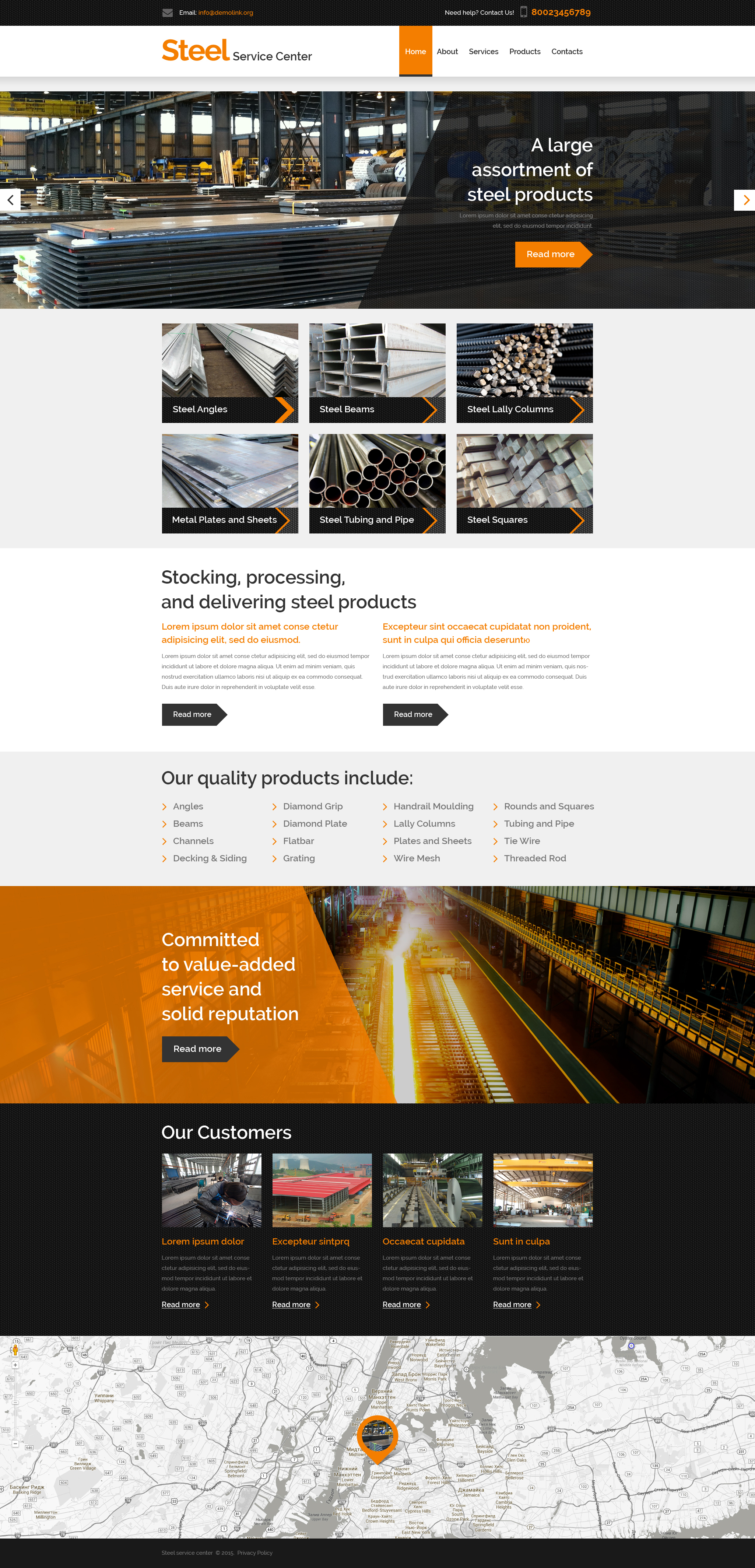Screenshot of a Steel Service Center Website

At the top of the screenshot, the header reads "Steel Service Center," with "Steel" in bold orange letters. The navigation bar includes the options: Home (selected), About, Services, Products, Contacts, and "Need help? Contact us" with a phone number 800-234-56789.

Below the header, there is a prominent photograph of a steel manufacturing plant with a caption that reads "A Large Assortment of Steel Products." Underneath, there is placeholder Latin text (Lorem Ipsum) accompanied by an orange arrow labeled "Read More."

The page showcases several images of steel products with corresponding labels beneath each:
- "Steel Angles" beneath a picture of steel angles
- "Steel Beams" beneath a stack of steel beams
- "Steel Lolly Columns" beneath a photograph of steel lolly columns
- "Steel Plates and Sheets" beneath a stack of metal sheets
- "Steel Tubing and Pipe" beneath a photograph of steel tubing and pipes
- "Steel Squares" beneath a photograph of steel squares

A section below features additional placeholder Latin text with black arrows labeled "Read More." It highlights the range of quality products available, including:
- Angles
- Beams
- Channels
- Decking and Siding
- Diamond Grip
- Diamond Plate
- Flat Bar
- Grating
- Handrail Molding
- Lolly Columns
- Plates and Sheets
- Wire Mesh
- Rounds and Squares
- Tubing and Pipe
- Tie Wire
- Threaded Rod

Another section emphasizes the company's commitment to value-added service and its solid reputation, followed by a "Read More" prompt.

The "Our Customers" section features photographs of steel plants with more placeholder Latin text beneath them.

At the very bottom of the screenshot, there is a map displaying an orange location pin, presumably indicating the company's location.